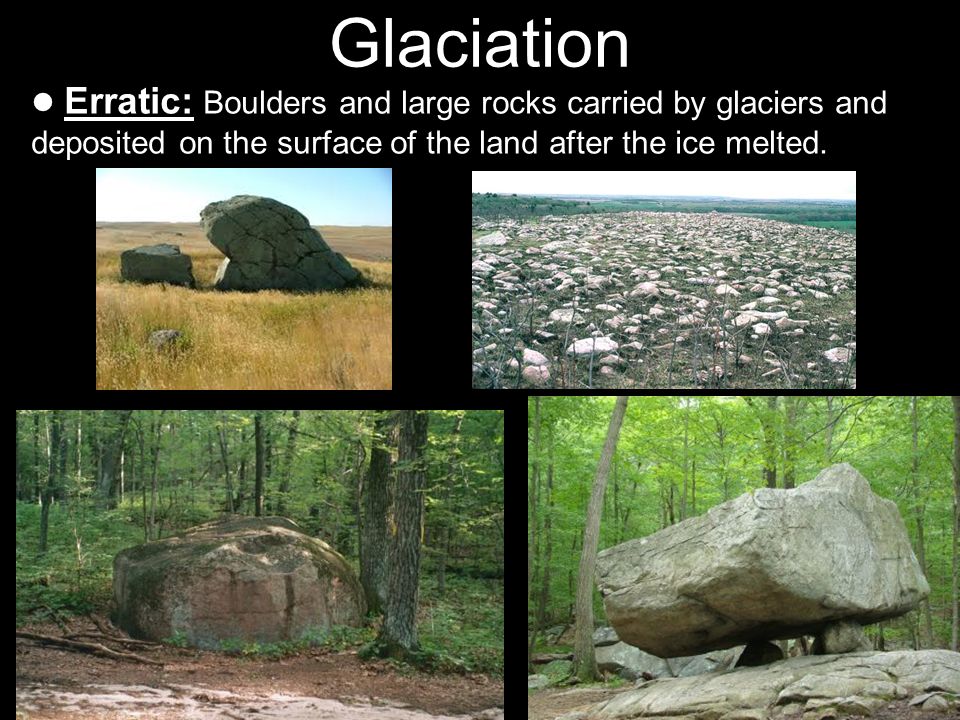The image features a black background with a prominent title in white letters that reads "Glaciation." Below the title, the term "Erratic" is highlighted with an underline. Accompanying this text is an informative statement: "Boulders and large rocks carried by glaciers and deposited on the surface of the land after the ice melted." The image displays four photographs, each showcasing different scenes of these glacial erratics. The upper left photograph captures two large rocks situated in what appears to be a field. The upper right image depicts a rocky landscape under a cloudy sky. The bottom left displays a massive boulder beside trees in a forested area, while the bottom right also features a large boulder amidst forest scenery, emphasizing the varied environments where these erratic rocks have been deposited by glaciers.